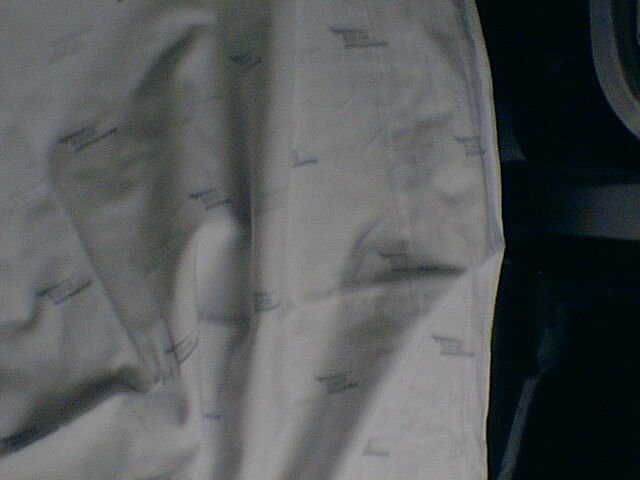The image depicts a close-up view of a crumpled, light-colored fabric, likely white or gray, placed against a dark background. The fabric appears to be soft and easily wrinkled, featuring numerous creases and folds that create shadows and emphasize its texture. Scattered across the fabric are small, almost square symbols or patterns, uniformly spaced in a zigzag arrangement. These symbols, possibly logos or lettering in black or blue, repeat consistently throughout the material. To the lower left of the fabric, there is a hint of what might be a pocket, suggesting the fabric could be part of a garment like a shirt or jacket. The dark background provides little clarity, though some silver-edged items are faintly visible, potentially indicating kitchen appliances or silverware, but their exact nature remains ambiguous due to the grainy and blurry quality of the photo.